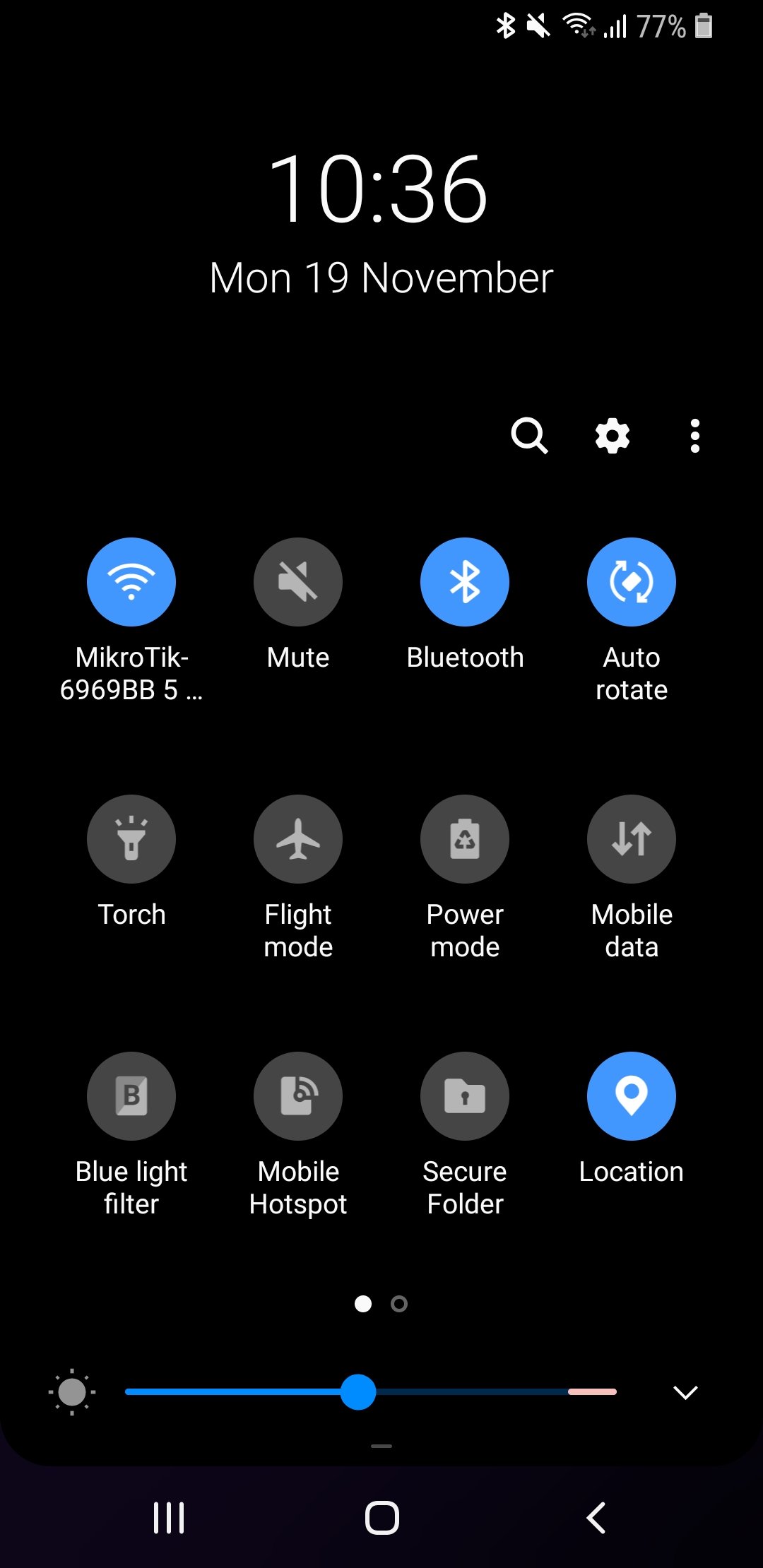The image features a close-up of a smartphone screen, emphasizing the detailed layout and various icons displayed. In the upper right corner, several status indicators are visible, including those for Bluetooth, cellular connection, Wi-Fi signal, and battery life displaying at 77%. The time "10:36" is prominently shown, along with the date "Monday, 19 November."

Below this, two icons—a magnifying glass for search and a gear for settings—are situated. The screen further displays rows of circular icons, each representing different functions.

On the top row, starting from the left, there is a blue circle icon labeled "Microtech 6969BB5..." followed by a dark gray circle with a microphone icon that has a line through it, indicating mute. Next, a blue circle with the Bluetooth logo labeled "Bluetooth," and an icon for auto-rotate.

The second row features a dark gray circle labeled "Torch," followed by a plane icon for "Flight Mode," a power-saving icon labeled "Power Mode," and a data icon with an upward and downward arrow labeled "Mobile Data."

The third row begins with a blue light filter icon, followed by an icon labeled "Mobile Hotspot," another for "Secure Folder," and a location icon highlighted with a blue background.

At the bottom, there's a brightness adjustment slider, depicted by a sun icon, halfway across the screen with a blue dot for adjustment. Below this slider are icons for navigation: three vertical lines representing the menu, a square icon for home, and an arrow pointing left for back navigation.